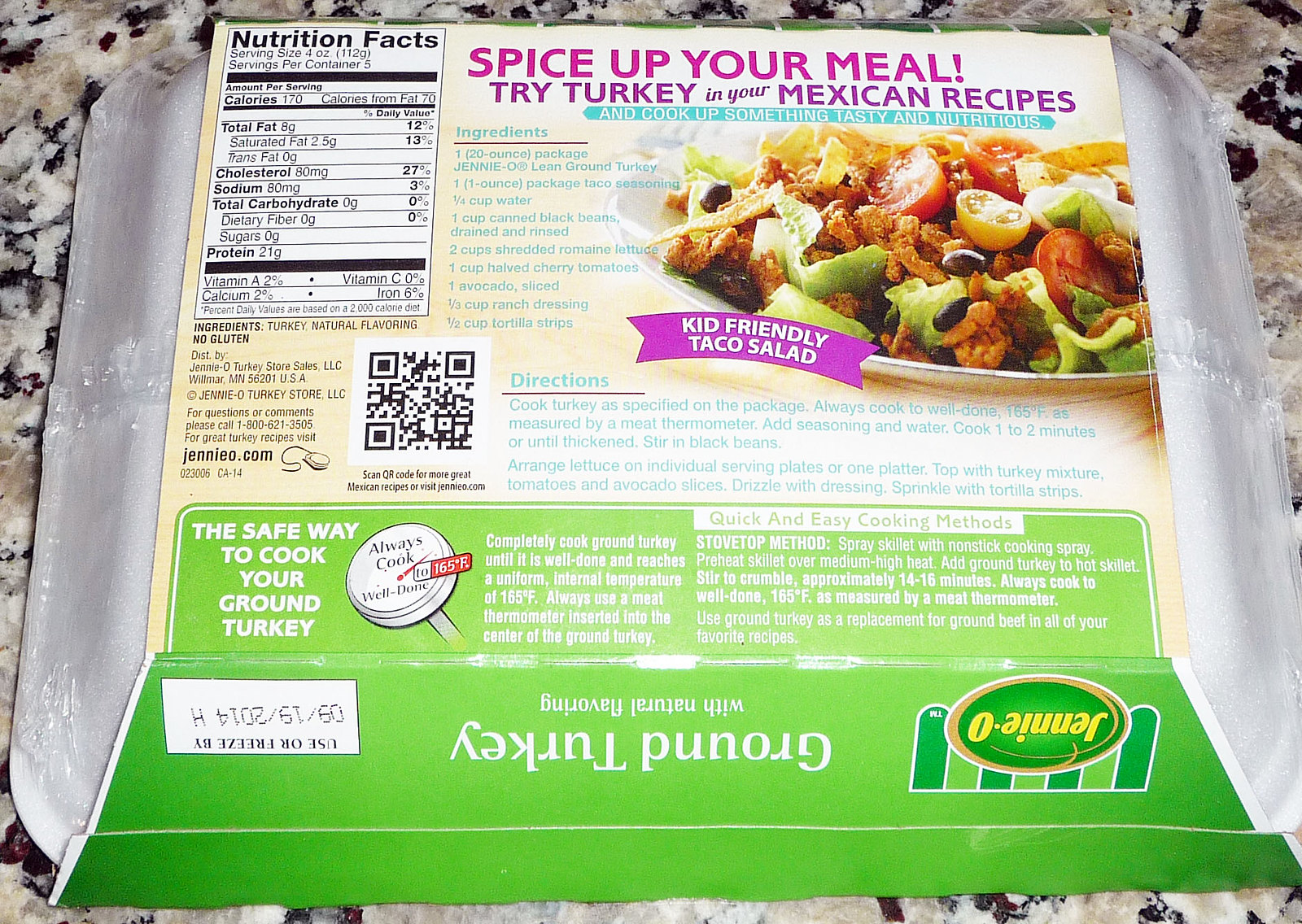This image depicts the backside of a ground turkey package from Jenny O, featuring comprehensive nutritional information, cooking instructions, and meal suggestions. The package is placed on a grey and black flooring, and it consists of a green and yellow bottom section with white sides. The nutritional facts are prominently displayed in the upper left-hand corner, featuring details such as serving size (four ounces), servings per container (five), and key nutrients like calories (170 per serving) and protein (21 grams).

Centered prominently is a recipe section urging consumers to "spice up your meal" by incorporating turkey into Mexican dishes, highlighted in red letters. Below it, a colorful image showcases turkey and vegetables on a white plate, alongside a fabric-like purple banner that reads "kid-friendly taco salad" in white text. The packaging also includes a green box specifying the safe cooking guidelines for ground turkey, featuring an icon of a turkey baster and instructions to always cook it well done. 

On the right side of the package, a Quick Response (QR) code scanner is visible, along with a bar code. The company name, Jenny O, appears at the bottom in an orange circle set against a green background with cascading light and dark green half-circles. These elements collectively provide a visually rich and informative look at the product, highlighting its safety, nutritional value, and versatility in meal preparation.